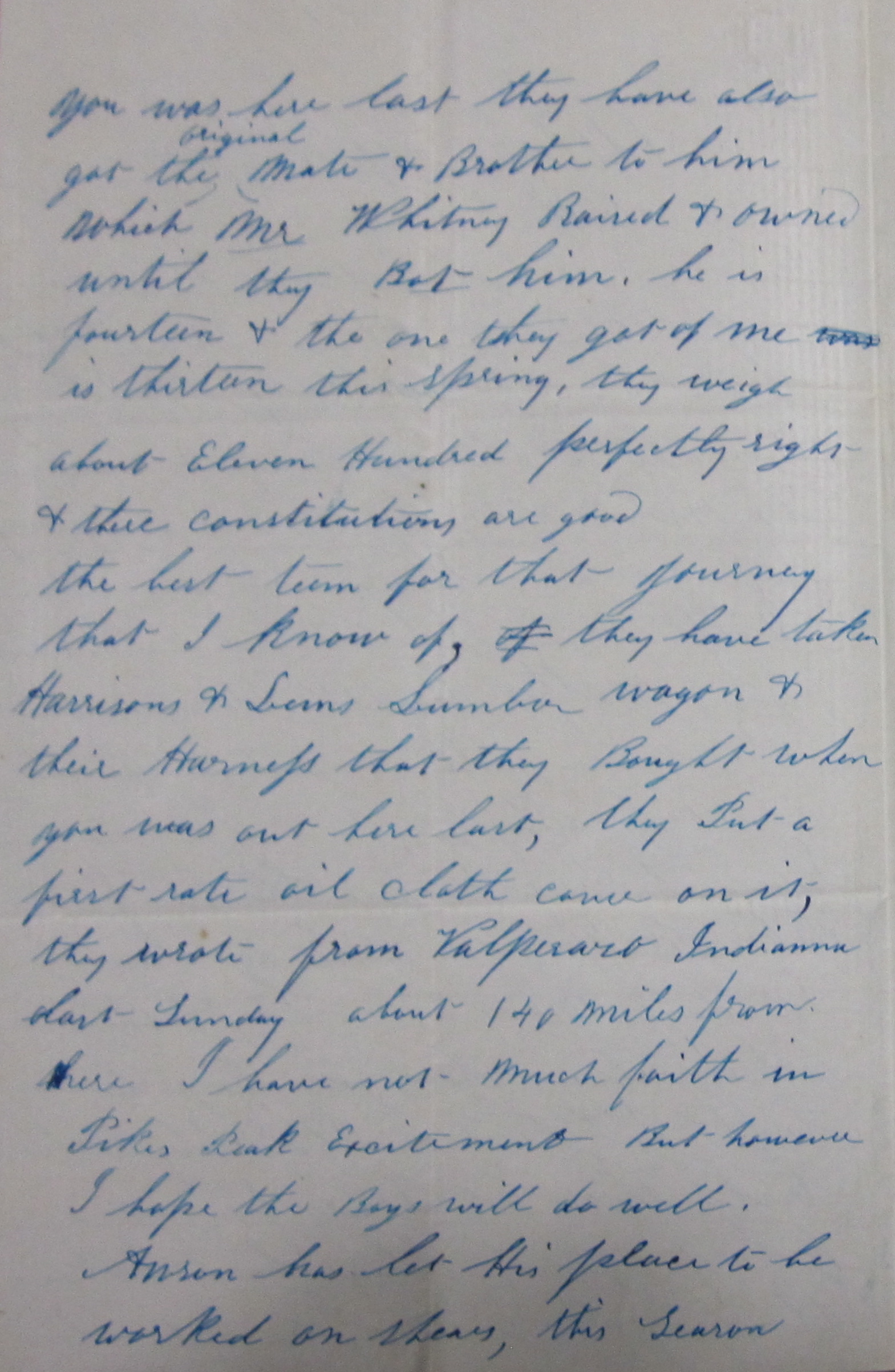The image portrays a handwritten letter in cursive, composed in blue ink on white paper that shows distinct fold lines, suggesting it was folded for sending. Despite some crossed-out mistakes, the writing is mostly neat cursive. The letter appears to be spread across three paragraphs, occupying most of the page from top to bottom. The contents are somewhat difficult to decipher, owing to both the personalized, stylized nature of the cursive and the image sizing, rendering parts of it illegible. The paper also looks slightly discolored or faded. The visible text includes fragments such as "you were here last night," mentions of "mate" and "brother," and seems to reference a journey involving a wagon, possibly covering about 140 miles. This detailed and somewhat indistinct writing hints at a personal narrative or historical correspondence.